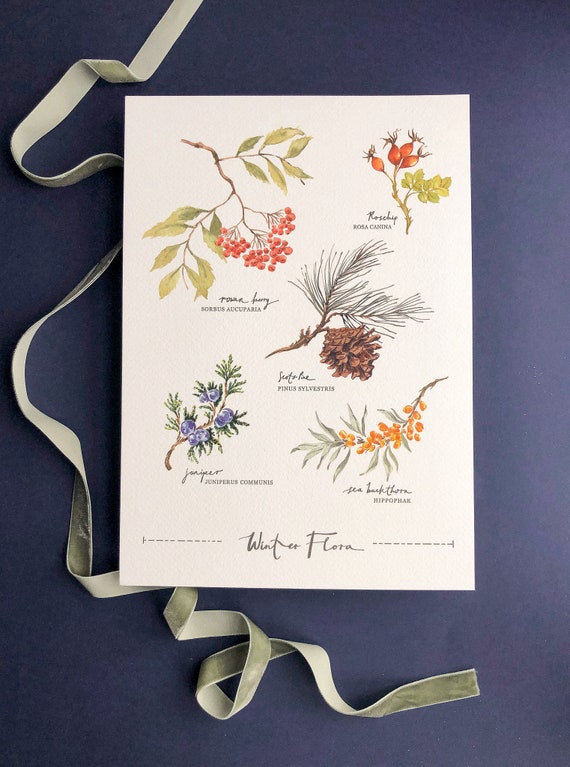The photograph features a rectangular card on a dark blue background, presenting detailed scientific illustrations of five different types of flora labeled as "Winter Flora" at the bottom center. The card displays varied flora, with colors including orange, brown, lavender, and lighter orange. The top left illustration depicts a twig with approximately 40 red berries and leaves. The top right shows a plant resembling a large radish with its leaves and root. The center features a pine cone and its distinctive leaves. The bottom left illustrates juniper, showing blueberries accompanied by fern-like leaves. The bottom right exhibits a plant with thin leaves and orange petals. A light gray ribbon is placed to the left and bottom of the card, and there is additional text around the "Winter Flora" label, though it is too small to decipher.